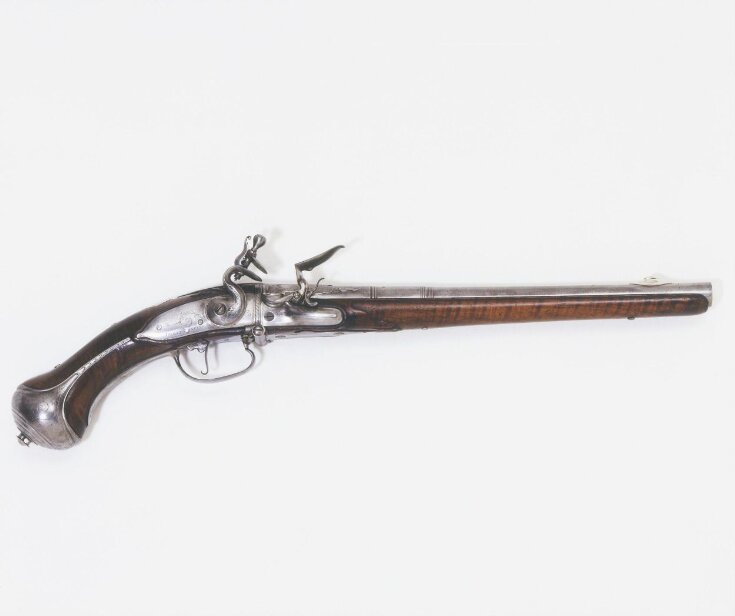This photograph captures a meticulously maintained, historical firearm set against a plain white background. The gun, which appears to be an old-fashioned musket or possibly an antique shotgun, boasts a distinctive, lengthy barrel. The barrel is a blend of polished silver, likely nickel-plated, and finely crafted brown wood at the bottom. The handle shares this dual-material design, with intricate silver plating and wooden detailing. The handle features a round cap with a small protruding knob, adding to its vintage aesthetic. A delicately crafted, thin silver trigger extends from the handle, adding to the gun's historical charm. Adjacent to the trigger is a silver apparatus, potentially the bullet chamber, adorned with latches and clasps that speak to the gun's antique engineering. The firearm is oriented with its barrel pointing to the right, and its pristine condition suggests it is either expertly preserved or displayed in a museum-like setting, free from any visible damage or wear.